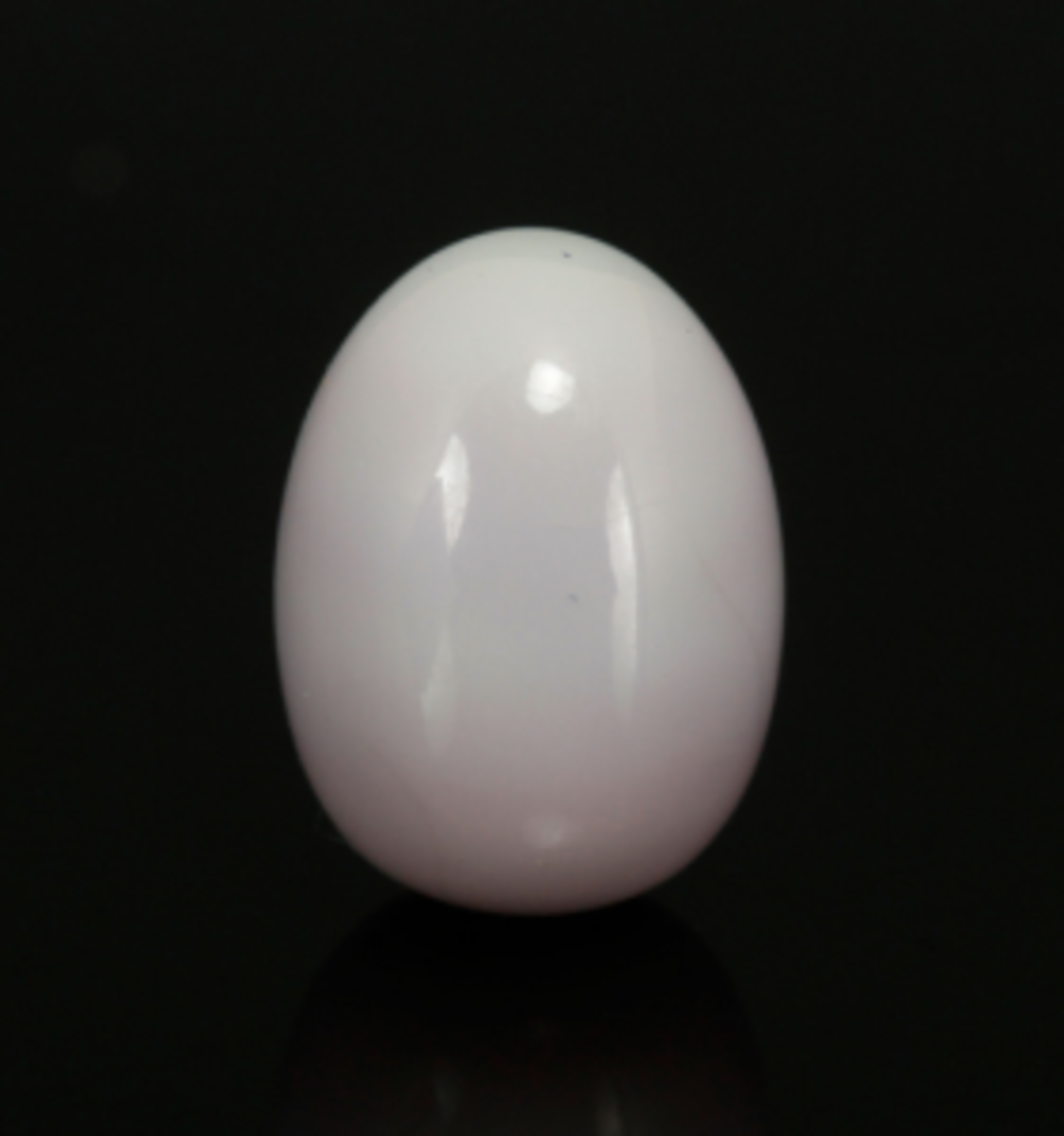The image presents a highly polished, oval-shaped object resembling an egg, set against a stark black background. The object, possibly made of a glossy ceramic or a shiny man-made material, reflects light on its smooth surface, accentuating its egg-like shape. At the very bottom of the image, a reflection of the object can be seen, reinforcing the impression of a shaded, black setting. The 'egg'—free of any significant markings or blemishes save for a few very light gray spots—appears flawless and pristine, standing upright in a simple, minimalist composition.